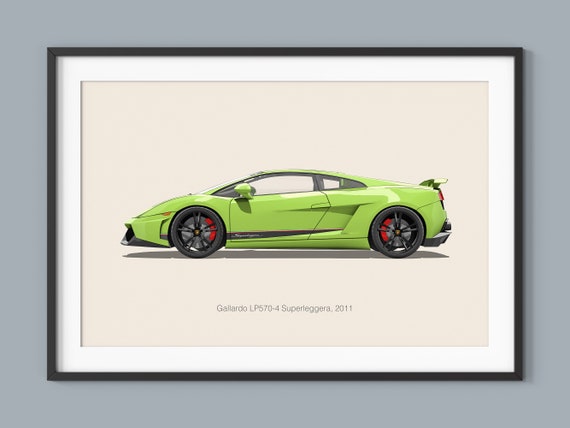This is a framed portrait of a lime green sports car, specifically identified as the Gallardo LP570-4 Superleggera 2011. The picture is elegantly encased in a black frame with a thinner black border followed by a thicker white border, set against an off-white background. The entire framed image is mounted on a somewhat dark gray wall, providing a contrasting backdrop that highlights the framed picture. The sports car is depicted from the driver's side, revealing detailed features such as a low front hood, a sleek profile with numerous indentations and lines that suggest speed, and a prominent rear spoiler. The car's wheels are a combination of black and brushed steel, showcasing red brake calipers. Black trim details accentuate the car’s body, including a line across the bottom where the model name is inscribed. This detailed image captures the essence of the high-performance vehicle, combining visual appeal with descriptive elegance.